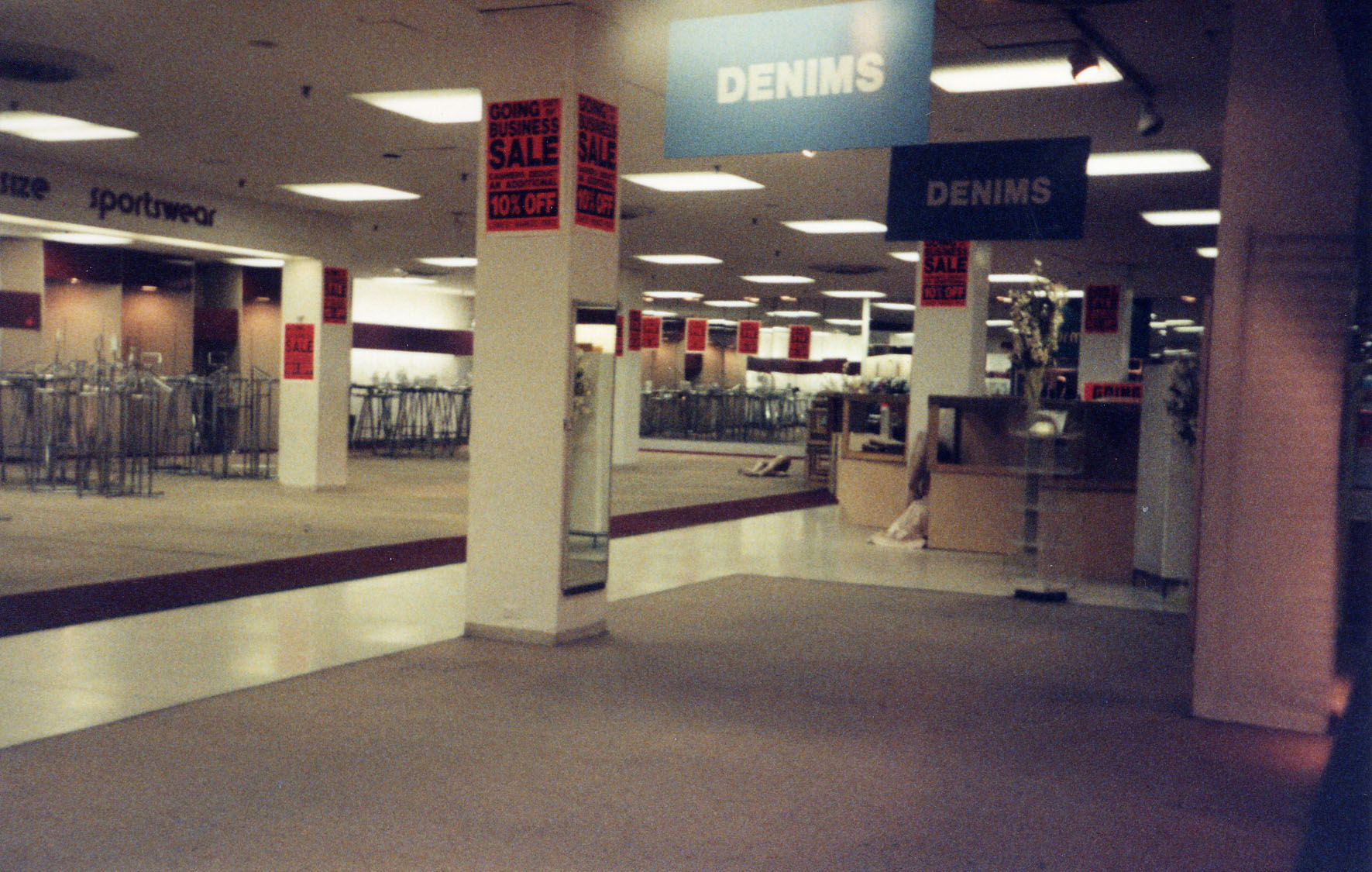This image depicts the interior of an almost empty department store's clothing section. The scene is dominated by numerous empty clothing racks scattered throughout the background, creating an overall desolate atmosphere. 
Suspended from the ceiling are various signs indicating different sections, including a prominent blue sign for 'Denim' and another for 'Sportswear' visible to the left. Columns standing throughout the floor are adorned with bright red sale signs, further suggesting a clearout or end-of-season sale is in progress. The store, designed with wide aisles and high ceilings, appears expansively vacant, drawing attention to the sparse arrangement of merchandise and the significant lack of customers.